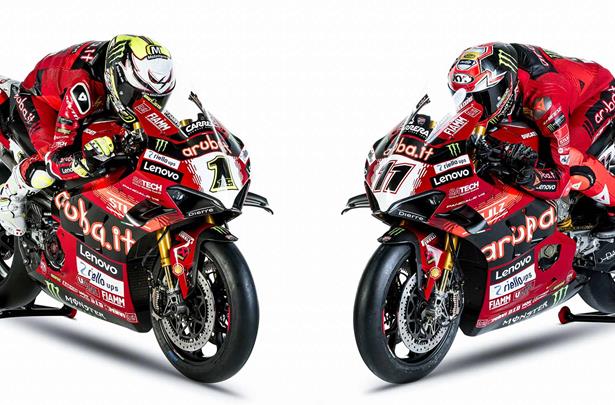This photograph features two racing motorcycles with riders, positioned on stands, facing each other in a V-formation against a white background. Both motorcycles are predominantly red, adorned with various sponsor logos such as Lenovo, Aruba, and potentially others like Zillow Apps and Cobalt. The bike on the left displays the number 7, while the bike on the right has the number 11. Each rider is wearing a coordinated red racing suit with different helmet designs— the rider on the right has a black helmet with red, white, and yellow accents, and the rider on the left sports a white helmet with black and yellow details, featuring a monster logo. Both bikes and riders are poised in a forward-leaning position, giving a dynamic sense of readiness and motion. The image emphasizes the heavily branded nature of professional racing bikes and gear.